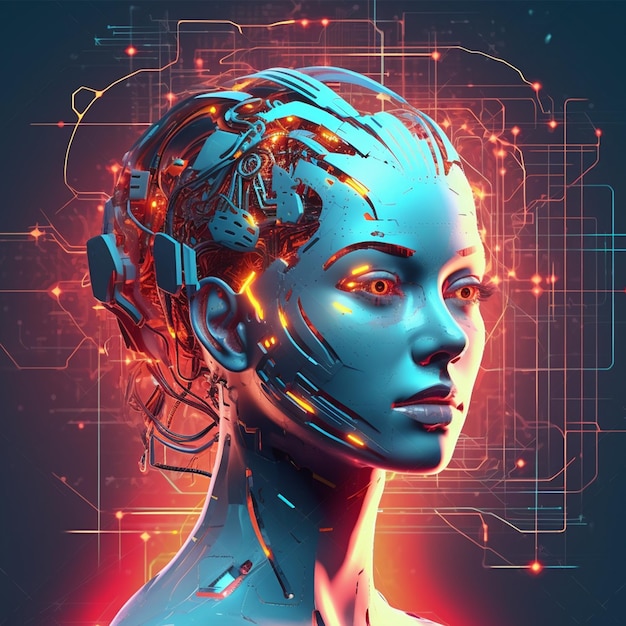This futuristic, computer-generated 3D image features the head of a female robot, designed with a metallic, medium blue turquoise finish. She faces toward her left, gazing straight ahead with glowing amber eyes that possess black centers. Her lips, full and closed, add to her humanoid appearance. The back of her head is open, revealing a complex array of bright wires and illuminated structures emerging, giving the impression of an exploding or disintegrating skull. These elements extend into a dark background adorned with a network of digital lines in various colors, including blues, reds, and oranges, punctuated by glowing dots of light. The strong illumination from the right side casts parts of her neck, shoulder, face, and brow in a near-white light, accentuating her metallic luster. The detailed depiction of wires and nodes surrounding her head evokes the intricate design of a computer motherboard.